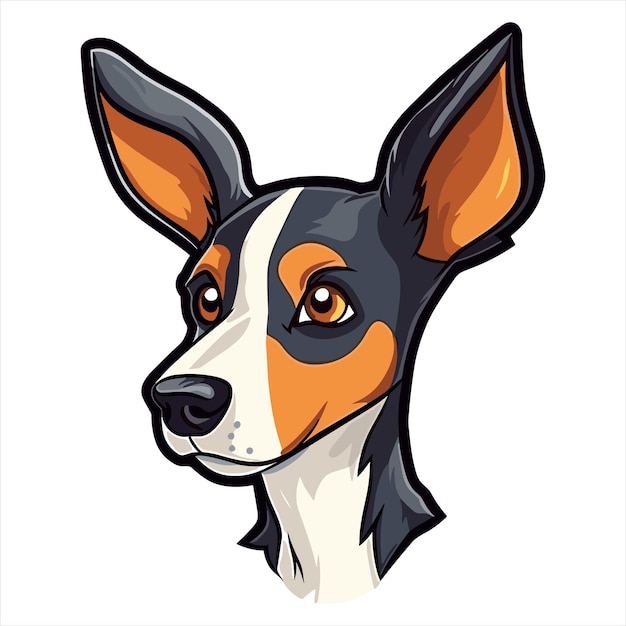This image portrays a detailed digital cartoon rendition of a dog's head and neck, resembling a Doberman. The dog features a narrow head and snout, with exceptionally large, pointed ears that are bordered by black outlines and internally colored with shades of orange and brown. The dog's face is primarily black with a distinct white stripe running from its nose, up its forehead, and down to the back of its head, continuing to its neck. The nose is black, surrounded by white, giving the appearance of a stripe. Bright brown eyes with orange accents and wide-open pupils convey an interested expression, looking off to the left. The dog's chin and under-neck areas are also white, contrasted by black sides. This finely crafted, cartoon-style illustration is both vibrant and expressive.